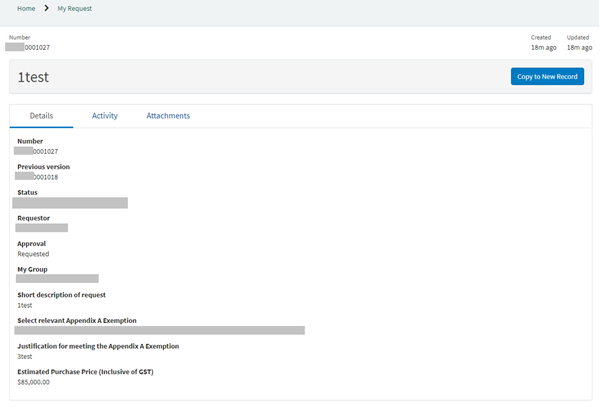The image is a horizontal screenshot of a web page featuring a thin, grayish top border. At the top left corner, there are navigation options labeled "Home," an "Arrow" icon, and "My Request." Below these, the page displays a label "Number" followed by a gray bar containing the number "0001027." To the right side of this gray bar, the timestamps "Created 18 minutes ago" and "Updated 18 minutes ago" are visible. Directly underneath is another light gray bar, which has the text "One Test" on the left and a blue button labeled "Copy to New Record" on the right.

Beneath these bars are three category headings: "Details," "Activity," and "Attachments." The "Details" tab is highlighted and marked by a light blue underline, while the words "Activity" and "Attachments" are displayed in blue text.

The "Details" section includes various elements:
- Number
- Previous Version
- Status
- Requester
- Approval
- My Group
- Short Description of Request
- Select Relevant Appendix A Exemption
- Justification for Meeting the Appendix A Exemption
- Estimated Purchase Price Inclusive of GST